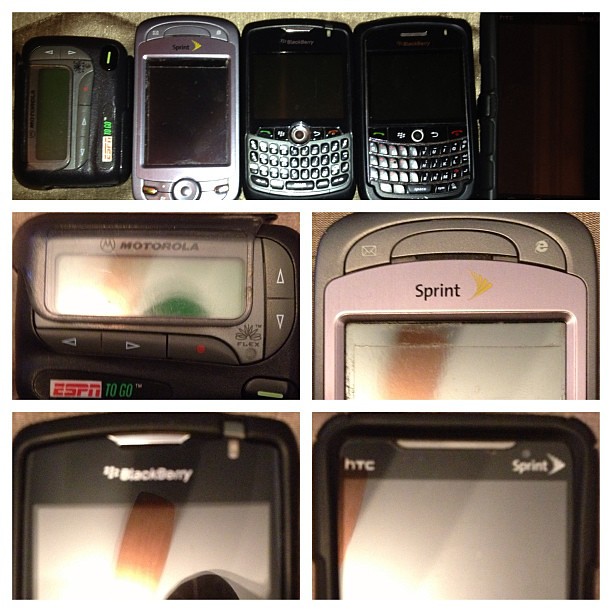The image is a detailed collage of five pictures showcasing vintage mobile devices, with one horizontal photo at the top lying across a grid of four close-up images beneath it. The top horizontal picture displays an array of old cell phones and a beeper, lined side by side. On the far left, a black beeper is visible, followed by a bulky phone resembling a tape deck marked with Motorola and an ESPN2Go logo. Nearby is a silver Sprint phone, two iconic BlackBerry devices with keyboards at the bottom, and an unspecified black phone on the upper right labeled HTC.

The four close-up images below provide intricate views of the devices in the top picture. The first close-up on the top left highlights the Motorola beeper with the ESPN2Go logo. Adjacent is a close-up of the silver Sprint phone, displaying the Sprint branding above the screen. The lower left close-up features a blurred BlackBerry phone, showcasing the BlackBerry name. Finally, the bottom right image captures the HTC phone, marked with Sprint on the right top corner. Each close-up emphasizes the unique features and branding of these nostalgic mobile devices.